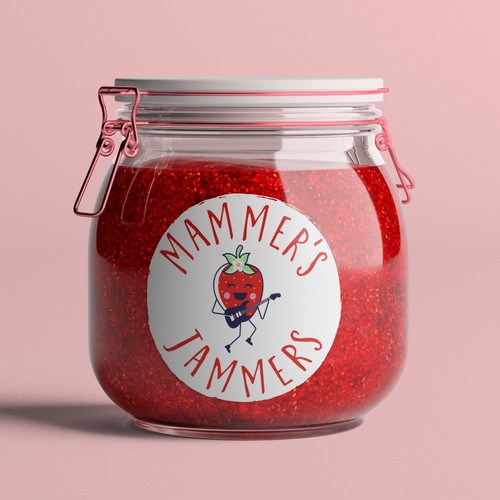The image presents a charming, squat, and round jar positioned directly at the center of the photo. The background is a solid, plain pink, highlighting the jar's details. The clear, see-through container, which appears quite fancy, contains a vibrant red mashed-up strawberry jam, speckled with tiny golden seeds. The jar is sealed with a white lid and fastened with a pinkish-red metal clasp. A white circular label with red uppercase text is attached to the front of the jar. The top of the label reads "Mammar's" and the bottom "Jammers." Between these words is a delightful illustration of a smiling strawberry stick figure playing an electric guitar, complete with arms, legs, and shoes. The overall setting and design suggest that this aesthetically pleasing jar might be featured on a specialty website dedicated to jams and jellies.